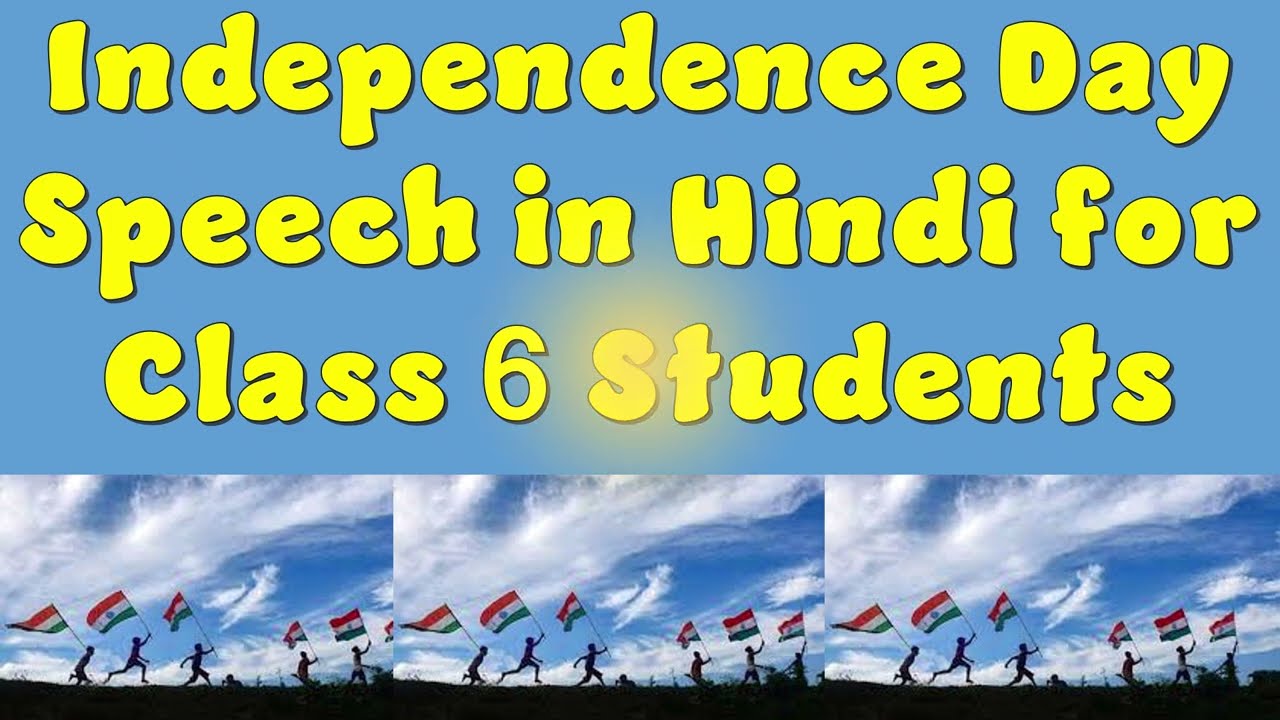The image has a landscape orientation and is divided into two main sections. The top three-quarters of the image features a blue background with yellow text displayed in three lines: "Independence Day," "Speech in Hindi for," and "Class 6 Students." A sun-like blemish or radiating light appears behind the "ST" in "Students," adding a subtle glow effect.

The bottom quarter of the image is divided into three identical photographs arranged horizontally. Each photograph depicts six children running with the Indian flag. The children are in various stages of sprinting, with the leftmost child slightly shorter than the two beside him, and the other children getting shorter towards the right. The Indian flag, which the children hold in their right hands, features a saffron stripe on top, a white stripe with a blue Ashoka Chakra in the middle, and a green stripe at the bottom. Behind them stretches a blue sky filled with scattered white clouds, providing a vibrant and dynamic background to the scene.